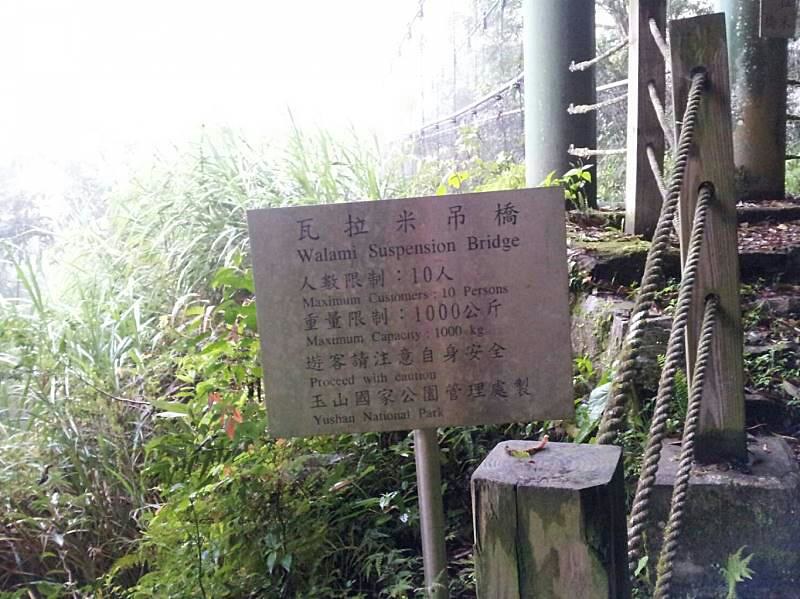This color photograph, taken in landscape orientation, captures a scene in an Asian national park, potentially Ushuari National Park. Dominating the image is a centrally positioned informational sign mounted on a silver post. The top of the rectangular metal sign features five Asian characters, likely Chinese, followed by English text that reads "Walami Suspension Bridge." The sign details that the bridge's maximum capacity is 10 persons and 1,000 kilograms. Below this are further instructions that translate to "Proceed with Caution" and the name "Ushari National Park." 

The right side of the image showcases a wooden staircase ascending towards the suspension bridge, flanked by a rope banister. The bridge itself is visible extending into the background, anchored by two light green pillars. On the left, the scene is framed by lush greenery, including trees, bushes, and various plants. There's a hint of hazy sunlight filtering from the top left corner, adding a natural highlight to the setting.